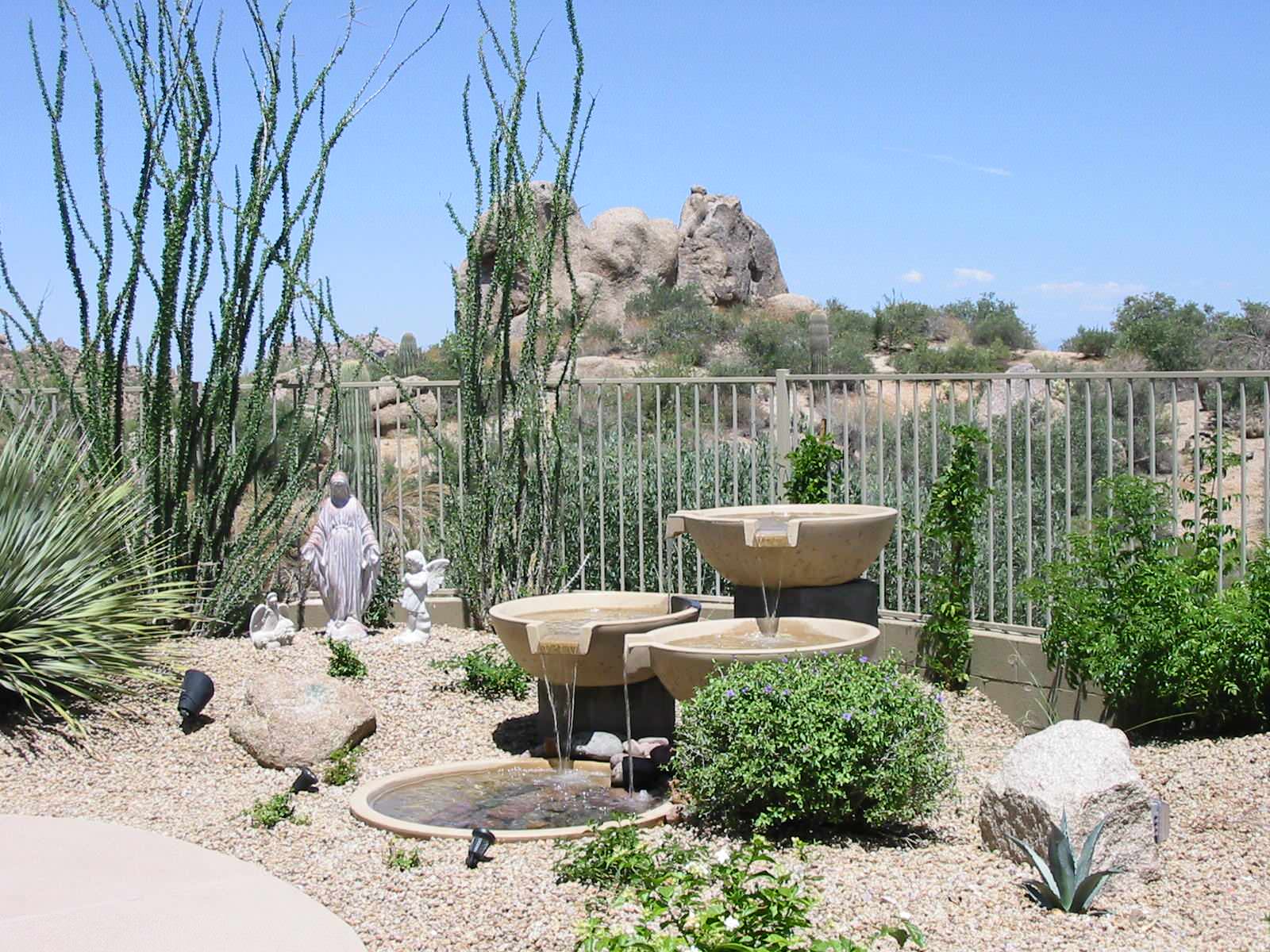This photograph captures a backyard garden situated in a desert or arid environment, accentuated by light gravel and dirt ground cover. The garden is enclosed by a beige metal fence and features a variety of green plants, including bushes and tall cacti, reflecting the arid region's vegetation. At the center of the image stands a three-tiered water fountain, where water cascades from the top bowl through to subsequent lower bowls, finally collecting in a small circular pit in the ground. Adjacent to the fountain on the left side, there is a black plastic garden light, and in the same area, a rock is visible. The background shows a faint trace of white wispy clouds against a bright blue sky, and far off are rock formations or mountain ranges with natural green shrubs. Additionally, the garden houses several religious statues, including two small angels and what appears to be the Virgin Mary, adding a spiritual touch to the scenic view.